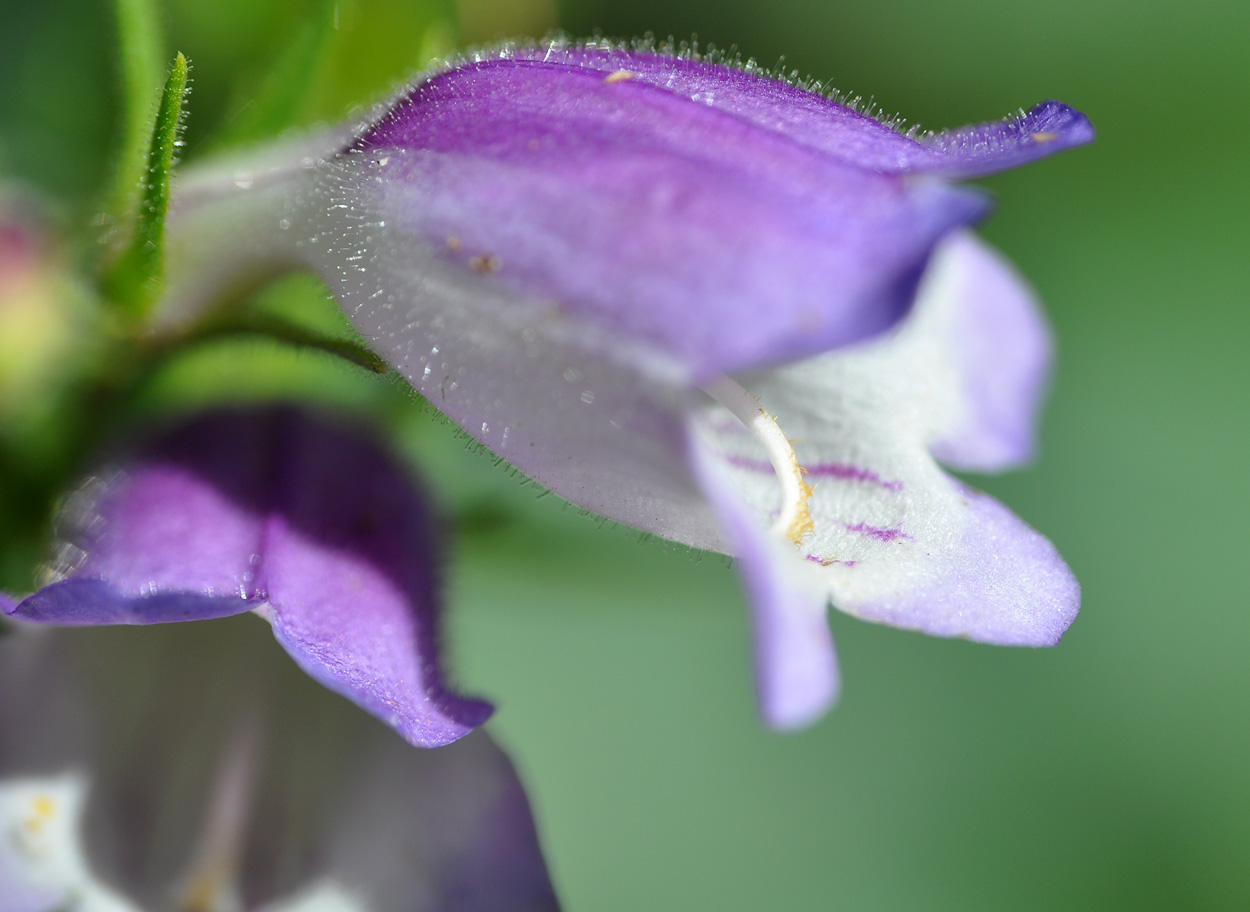This image showcases a high-definition, close-up view of a striking violet flower in full bloom. The flower exhibits a captivating combination of colors: its petals are primarily purple, varying from dark to light shades, while the interior features elegant white with delicate purple lines. Prominently emerging from the flower's center is a white stamen, tipped with a hint of yellow. To the lower left, another partially visible petal mirrors the same vivid purple hue. Surrounding the flower, green leaves and additional green floral elements peek through, suggesting new growth. The background, also green but slightly blurred, emphasizes the sharp detail of the flower itself. Tiny, silvery bristles can be seen on the top petal, adding to the intricate details of the photograph. Overall, the image highlights the flower's beauty against a natural green backdrop, illuminated by natural sunlight.